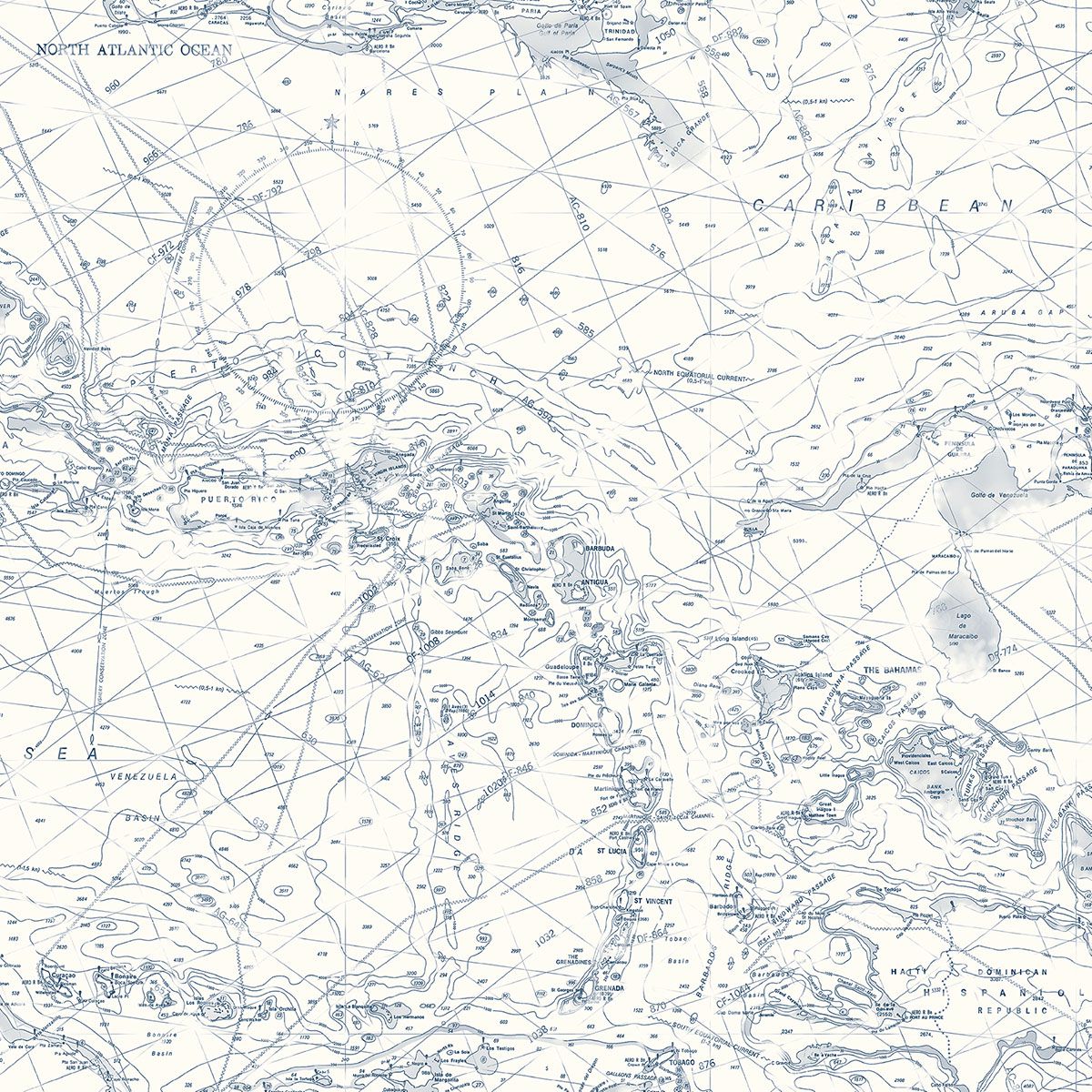This black-and-white, up-close, cross-sectional image appears to be a navigational chart or map. It details the North Atlantic Ocean and the Caribbean, with several continents and bodies of land and water intricately sketched. Key regions like Venezuela and Puerto Rico are marked, as well as the Dominican Republic in the bottom right. A compass is drawn in the middle, surrounded by a dense array of coordinate lines, navigational paths, and other chart markings, creating a complex and detailed composition. Despite its high level of detail, the image’s low quality makes the smaller text and numbers challenging to read, though prominent labels like "North Atlantic Ocean" and "Caribbean" are discernible. The illustration captures the essence of an old-fashioned maritime chart, used for navigating across oceans and seas.